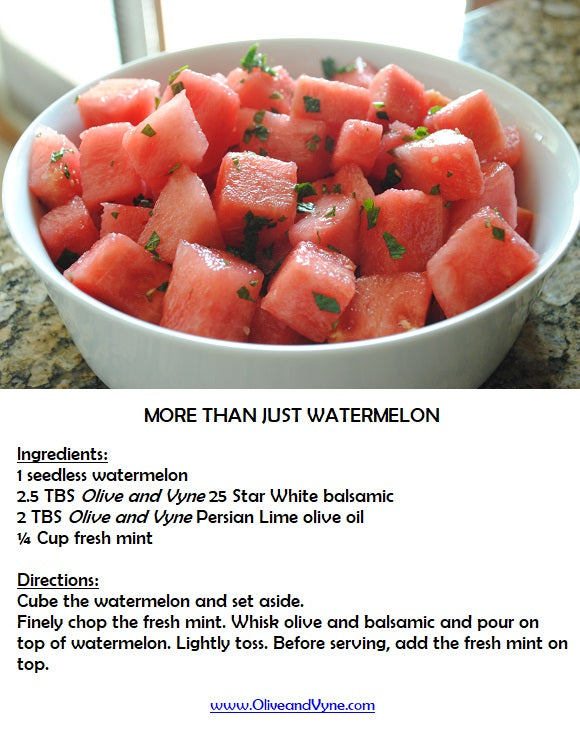This is a vertical rectangular printout featuring a refreshing watermelon recipe from Olive and Vine (www.oliveandvyne.com). The top section showcases a photograph of the prepared dish: cubed watermelon, lightly tossed with finely chopped fresh mint, and dressed with a mixture of olive oil and balsamic vinegar, all beautifully plated in a white serving dish on a countertop. Subtle greenery, potentially mint leaves, complements the vibrant red of the watermelon, hinting at the fresh ingredients used. Below the image is a bold title in large black text stating "More Than Just Watermelon." The text transitions into two main sections: Ingredients and Directions, each underlined for clarity. The Ingredients list includes one seedless watermelon, 2.5 tablespoons of Olive and Vine 25 Star White Balsamic, two tablespoons of Olive and Vine Persian Lime Olive Oil, and a quarter cup of fresh mint. The Directions succinctly guide the reader through cubing the watermelon, finely chopping the mint, whisking the olive oil and balsamic, pouring the mixture over the watermelon, and lightly tossing everything before adding the fresh mint on top. At the bottom of the page, the website for the recipe—www.oliveandvyne.com—is displayed in blue, underlined text.